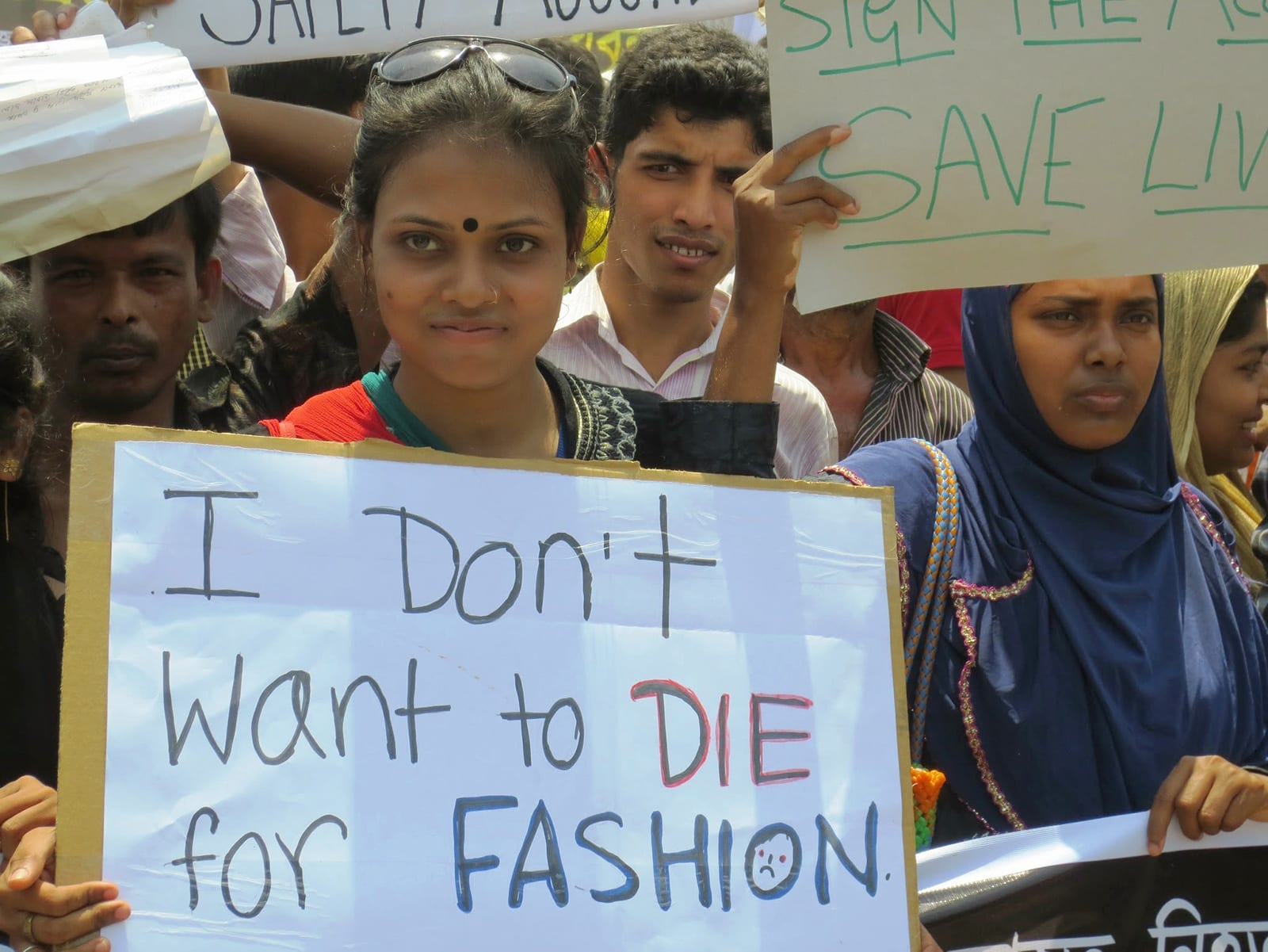The image captures a poignant, vibrant protest believed to be taking place somewhere in South Asia, possibly India. The demonstrators, likely low-wage garment workers, stand united in their plea for safer working conditions and better wages. At the forefront, a young woman with dark hair pulled back, a dark dot (bindi) between her eyes, and sunglasses perched on her head holds a prominent handmade sign with a cardboard backing. The sign, decorated with a sad face inside the "o" of "fashion," reads, "I don't want to die for fashion." Her shirt features multi-colored patterns in shades of orange, green, and black. To her right, another woman in a blue dress with a matching head covering clutches a sign advocating to "save lives." Several other demonstrators, some with headscarves and others without, hold up similarly handmade signs. Behind them, men and women stand in solidarity, some carrying items atop their heads. The protest occurs under bright sunlight, casting a serious, determined resolve across the faces of the participants, as they demand vital changes to their hazardous working environments.